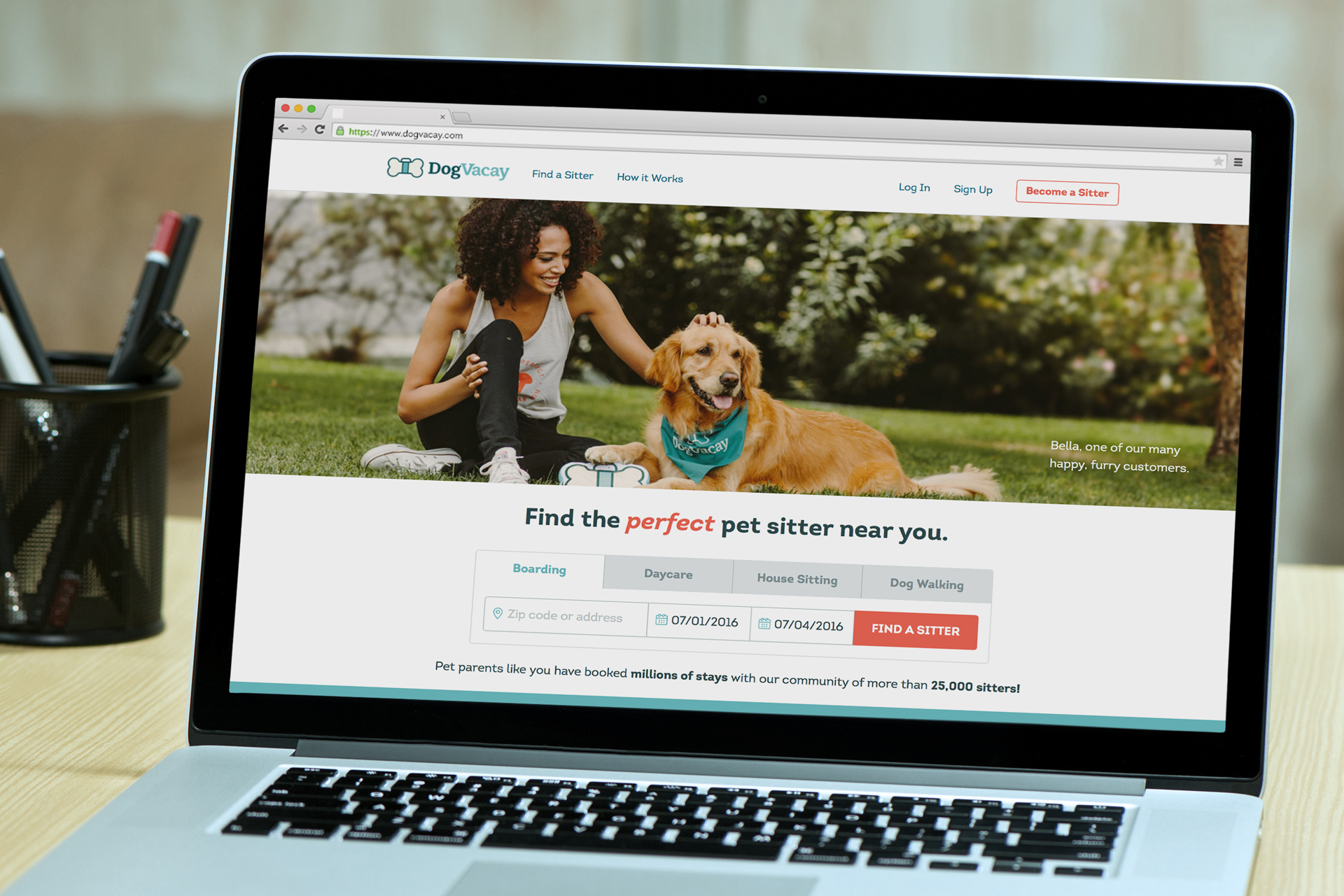A sleek laptop computer with a black screen border, silver base, and black keys sits atop a tan wood table. To the left of the laptop, there's a mesh metal cup holding several pencils. The background features a wall painted in a mix of tan and white. The laptop's screen displays an open web page for "Dog Vacay," which includes options to find a sitter, learn how the service works, log in, sign up, or become a sitter. The page highlights a photo of a woman crouched in the grass with a dog wearing a blue bandana, labeled as "Bella, one of our many happy furry customers." The site invites users to find the perfect pet sitter nearby, offering services such as booking boarding, daycare, house sitting, and dog walking. There are input fields for a zip code or address, dates of service, and a "Find a Sitter" button. Additionally, the page mentions that pet parents have booked millions of stays with a community of over 25,000 sitters.